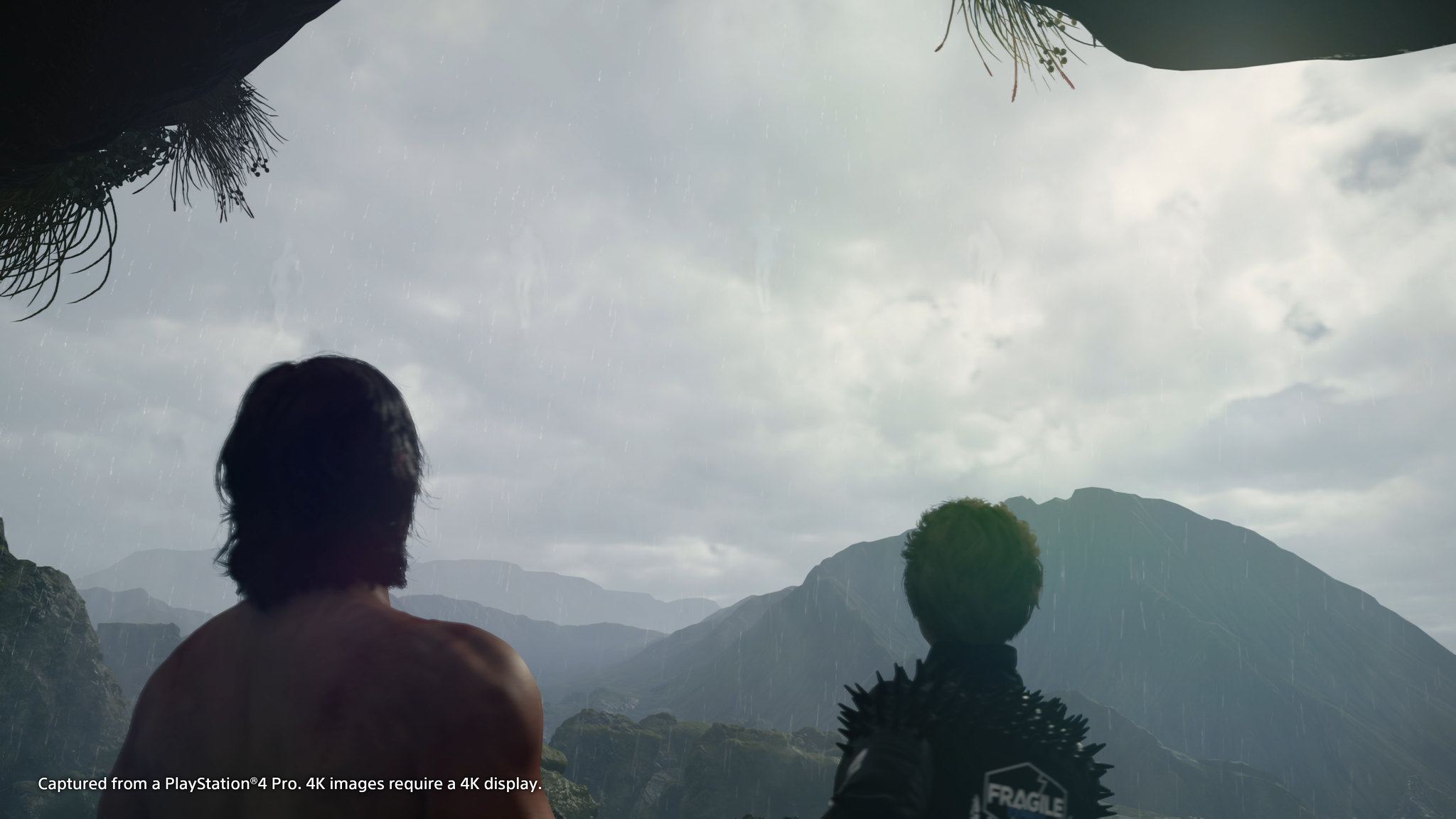In this captivating image, captured from a PlayStation 4 Pro, an inscription in the bottom left-hand corner informs viewers that 4K resolution requires a 4K display for optimal viewing. The scene features two individuals standing side by side, gazing intently into a majestic mountain landscape. 

On the left stands a shirtless figure with almost shoulder-length hair, exuding a sense of rawness and simplicity. Beside them, on the right, is another person, identifiable by a distinctive, short, curly hairstyle reminiscent of a small afro. This individual is clad in a striking, spiked black jacket emblazoned with the word "Fragile" across the back, adding an edgy and intriguing element to the scene.

The perspective offered in the image is exclusively from behind, revealing back views of these figures, including their heads, shoulders, and upper backs. This mysterious vantage point preserves the anonymity of the pair, drawing the viewer's focus towards the expansive and inviting mountainous vista that stretches out before them. The high level of detail and realism in the characters' appearances and attire makes it challenging to discern whether they are real people or exquisitely animated figures.